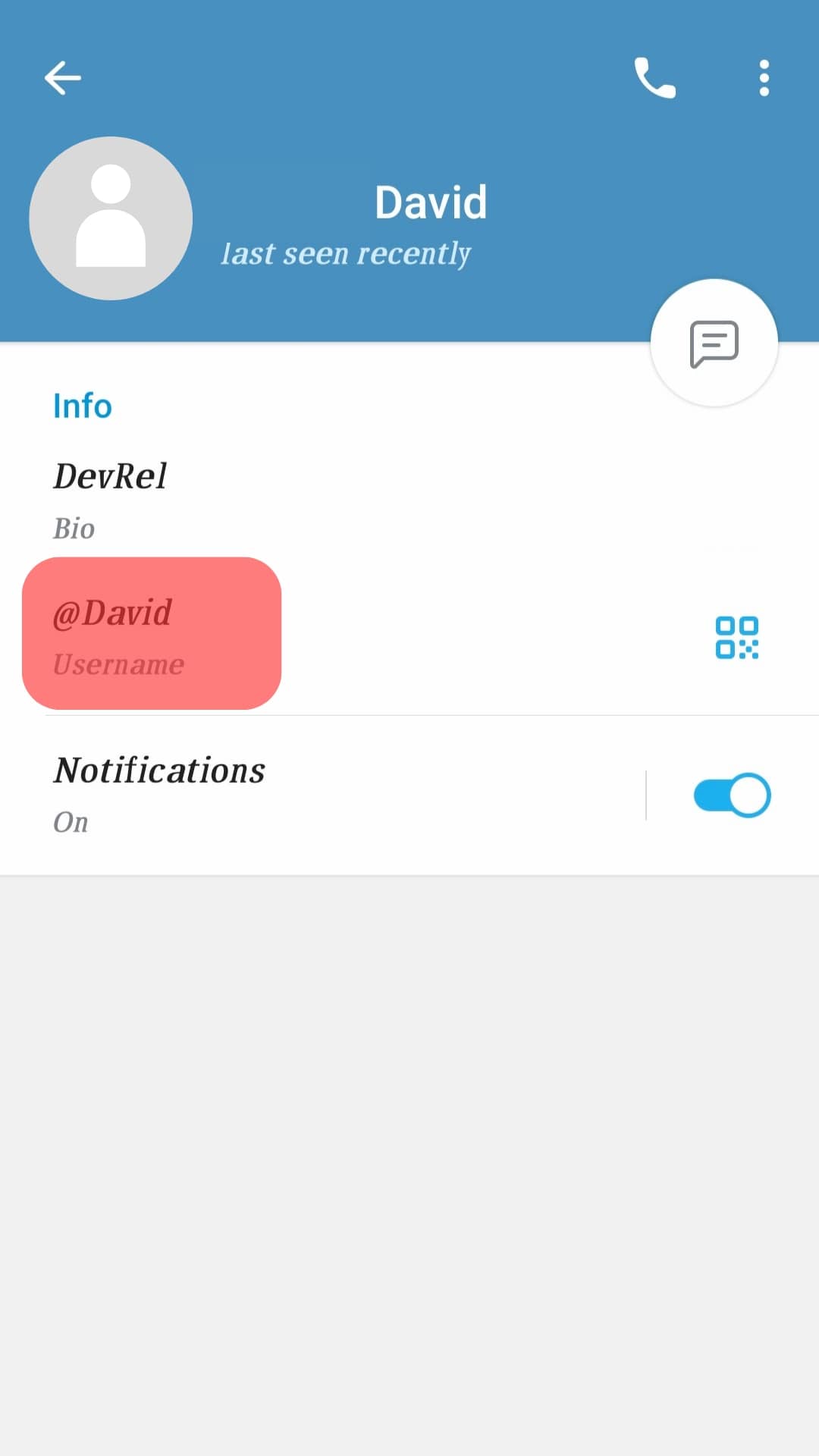The image depicts a user interface screen, possibly from a messaging or social media application. At the top of the screen, there's a blue header with a left-pointing arrow, a phone handset icon, and an ellipsis (...). Below the header, a gray and white generic default profile picture is displayed, along with the text "David last seen recently".

In the middle of the screen, there is a white oval containing a text box. Inside the text box, there's a blue "info" label, a black "devrel" label, followed by a gray "bio" label. Beneath this text box, there is a pink rectangular box labeled "@David username".

Further down, there's a section that reads "notification on", accompanied by a blue toggle switch set to the on position. To the left of the toggle switch, a small vertical line is visible, above which there is an unidentified blue icon.

Towards the bottom of the screen, a light gray rectangular area is present, currently filled with empty space.